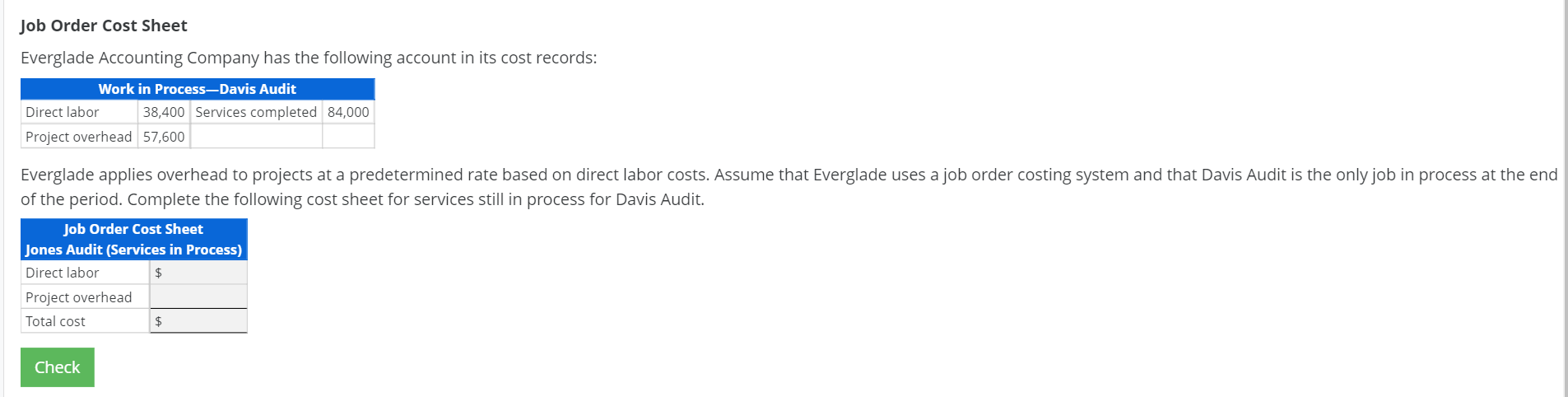**Caption:** 

The image appears to be a small section of a screenshot, likely from an accounting software or a job costing application, presented on a clean white background. In the upper left corner, the text "Job Order Cost Sheet" is printed in dark blue. Directly below, it reads, "Everglade Accounting Company has the following account and its cost records." 

A blue banner with white text, "Work in Progress - Davis Audit," seems to act as a heading for a table that follows. This table, consisting of two lines, lists the costs associated with the audit: 

- Direct Labor: $38,400
- Services Completed: $84,000
- Project Overhead: $57,600

Spanning the entire width of the image is a line of very small text, stating: "Everglade applies overhead to projects at a predetermined rate based on direct labor costs. Assume that Everglade uses a job order costing system and that Davis Audit is the only job in progress at the end of the period. Complete the following cost sheet for services still in process for Davis Audit."

Below this text is another table with a blue header labeled "Job Order Cost Sheet" and subtitled "Jones Audit, Parents, Services in Process." This table has blank spaces next to headings "Direct Labor," "Project Overhead," and "Total Cost," suggesting that these fields need to be filled in. 

To the right of the table, there's a green check button, which appears to be intended for submitting or confirming the entries. The rest of the screen content is aligned to the left side, leaving much of the white background uncluttered.